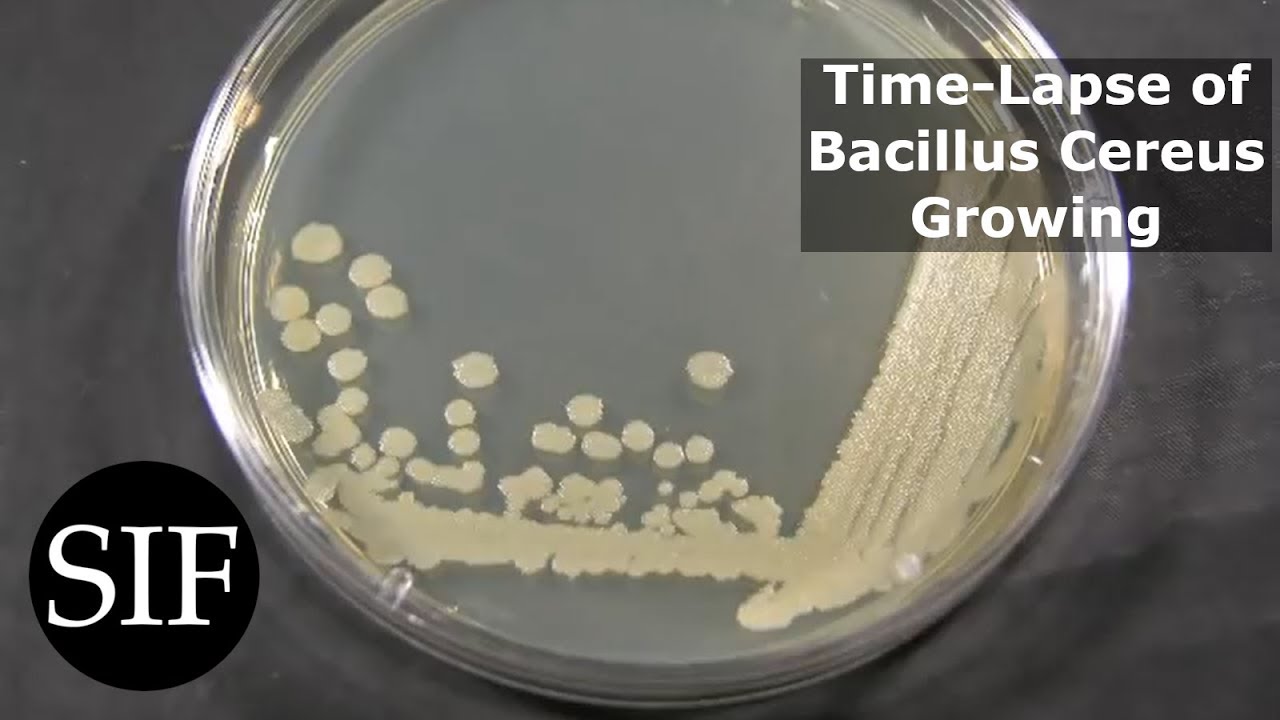The image depicts a scientific time-lapse of Bacillus cereus growing. It centers around a clear, circular Petri dish, which is placed against a gray, slightly bunched-up fabric background. Inside the Petri dish, the Bacillus cereus appears as various formations of off-white to pale yellow, with some gold-tinted areas. The left side of the dish features raindrop-like bacterial spots, while the right side showcases more linear streaks. Adding to the detailed description, a long gold streak runs along the bottom of the dish. At the lower left corner of the image, there's a black circle with the white uppercase letters "S-I-F," and on the upper right side, a lighter black rectangle is labeled with the white text "time-lapse of Bacillus cereus growing."